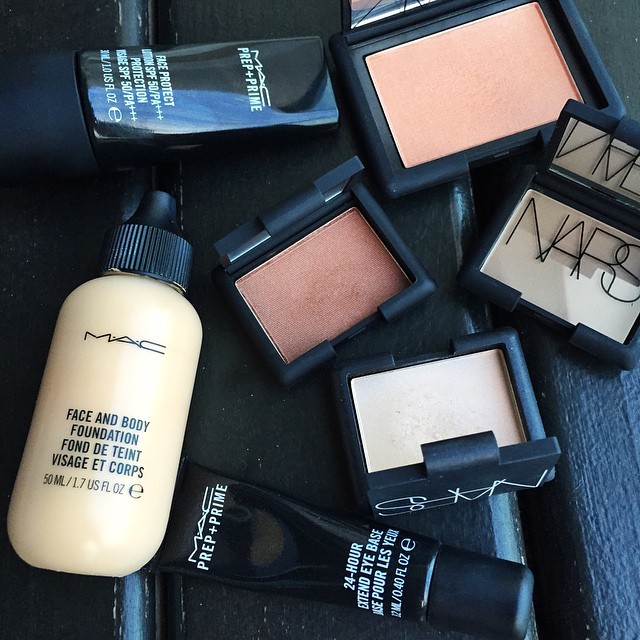The image displays an array of women's cosmetics methodically arranged on a surface made of dark wooden planks, which could either be a bench or table. At the top, there's a black tube labeled "Prep and Prime" from MAC. Adjacent to this is a trio of makeup shades in a square compact, featuring brown, darker brown, and tan or white colors. To the right of the trio is another square compact, and further left is a bottle with "MAC" inscribed on it, specifically detailing "Face and Body Foundation" in both English and French.

There are four cosmetic compacts of varying colors, one of which is from NARS, marked in white stylized letters. Scattered among these are several squeeze bottles. Notably, there are multiple tubes from MAC's Prep and Prime line, including a "24-Hour Extend Eye Base" and another labeled "Face Protect SPF 50."

In total, seven cosmetics items are spread out against the textured backdrop, providing a detailed overview of different makeup essentials.